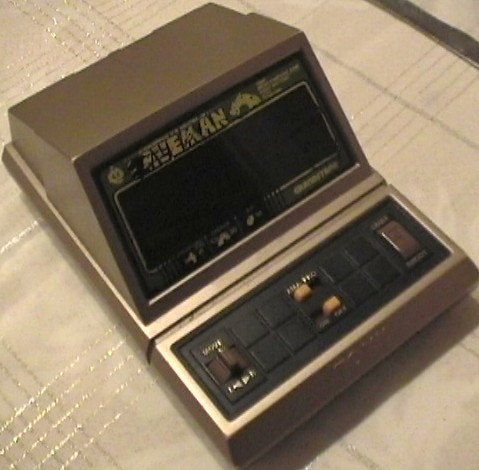This is a close-up photo of a somewhat blurry, old electronic device that has a vintage appearance, possibly from the late 70s or early 80s. The device is housed in a matte bronze casing with a black instrument plate set at a 45-degree angle. The top of the black faceplate contains indistinct and partially worn-off text, which might spell "Caveman" or something similar. At the bottom of the faceplate, there is a horizontal flat section featuring several buttons and potentially a small display, which is currently turned off. 

On the far left is a larger brown button labeled "Mode," followed by two smaller orange buttons in the middle that seem to slide side to side. On the right side, another button is present, though the text is also unreadable due to wear. The device gives off an impression of a potential old guitar effects pedal or a primitive gaming console, supported by intricate etched patterns on the beige tile background it rests upon. The device also shows a clear sign of age through its worn-out print and ambiguous features. The background is composed of off-white tiles with etched lines and a streak of dark gray in the upper right corner.